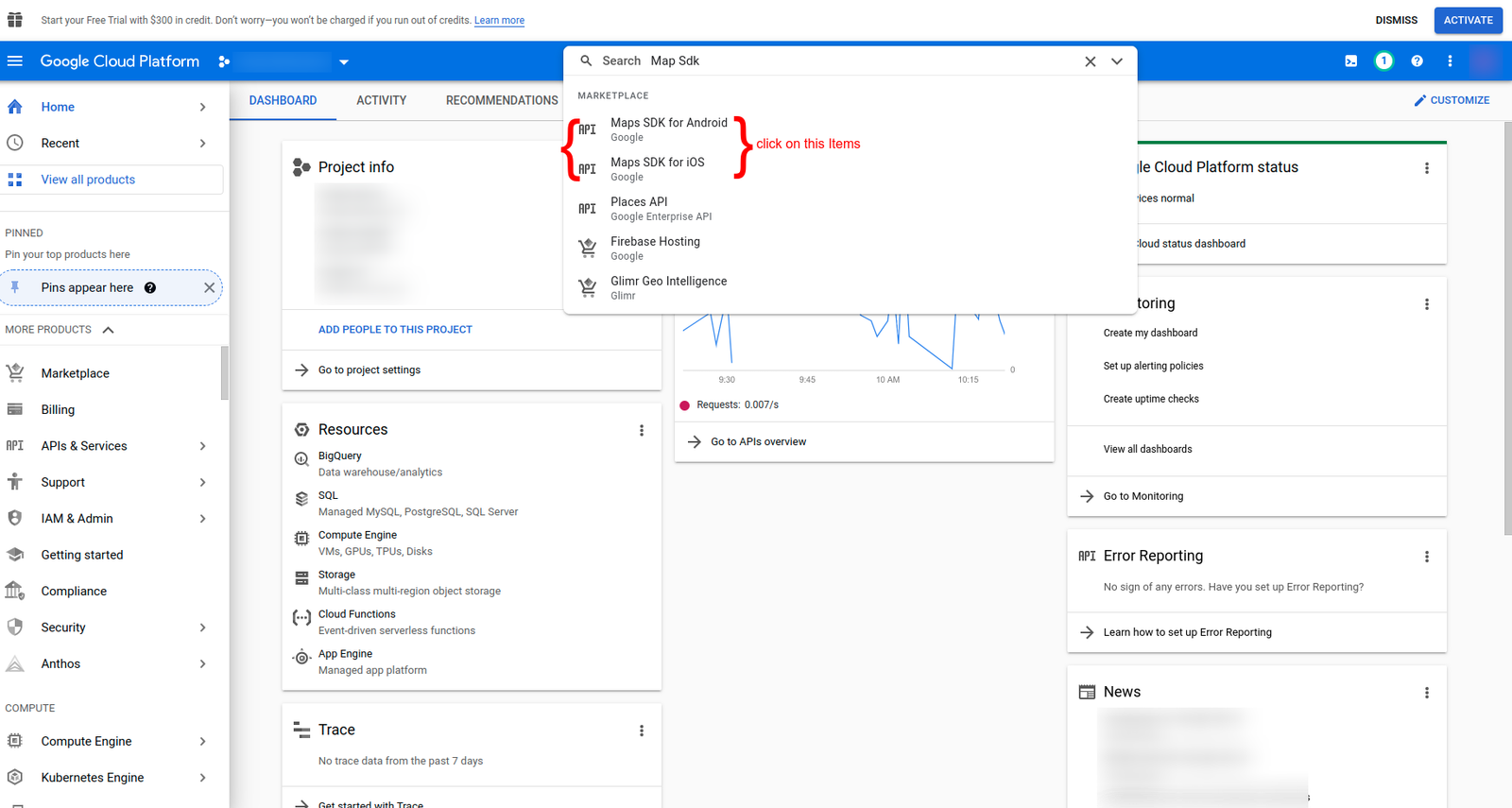This image captures the file structure interface of the Google Cloud Platform. The interface features a clean, predominantly white background with black and gray text. At the very top of the screen, a blue navigation bar displays the Google Cloud Platform logo, accompanied by an icon of three stacked lines (resembling pancakes or equal signs) on the left. To the right of the bar, there is a search bar and a few icons, along with options labeled "Dismiss" and "Activate" in the upper right corner.

The main navigation pane appears on the left side of the screen and includes several menu items such as "Home," "View All Products," "Marketplace," "Filing," "APIs and Services," "Support," "IAM and Admin," "Getting Started," "Compliance," "Security," "Authins," "Compute Engine," and "Code Engine." The section labeled "Pins Appear Here" sits just below the top menu items.

On the right side of the screen, the main content area showcases an ongoing search operation with the keywords "Map as Map" or "Manager SDK" highlighted. Below this, there are clickable items within parentheses. The content in this area is text-heavy and primarily composed of black and gray words, with a small graph embedded in the central region, adding a visual element to the text.

Overall, the interface provides a detailed view of the Google Cloud Platform's file structure and navigation elements.